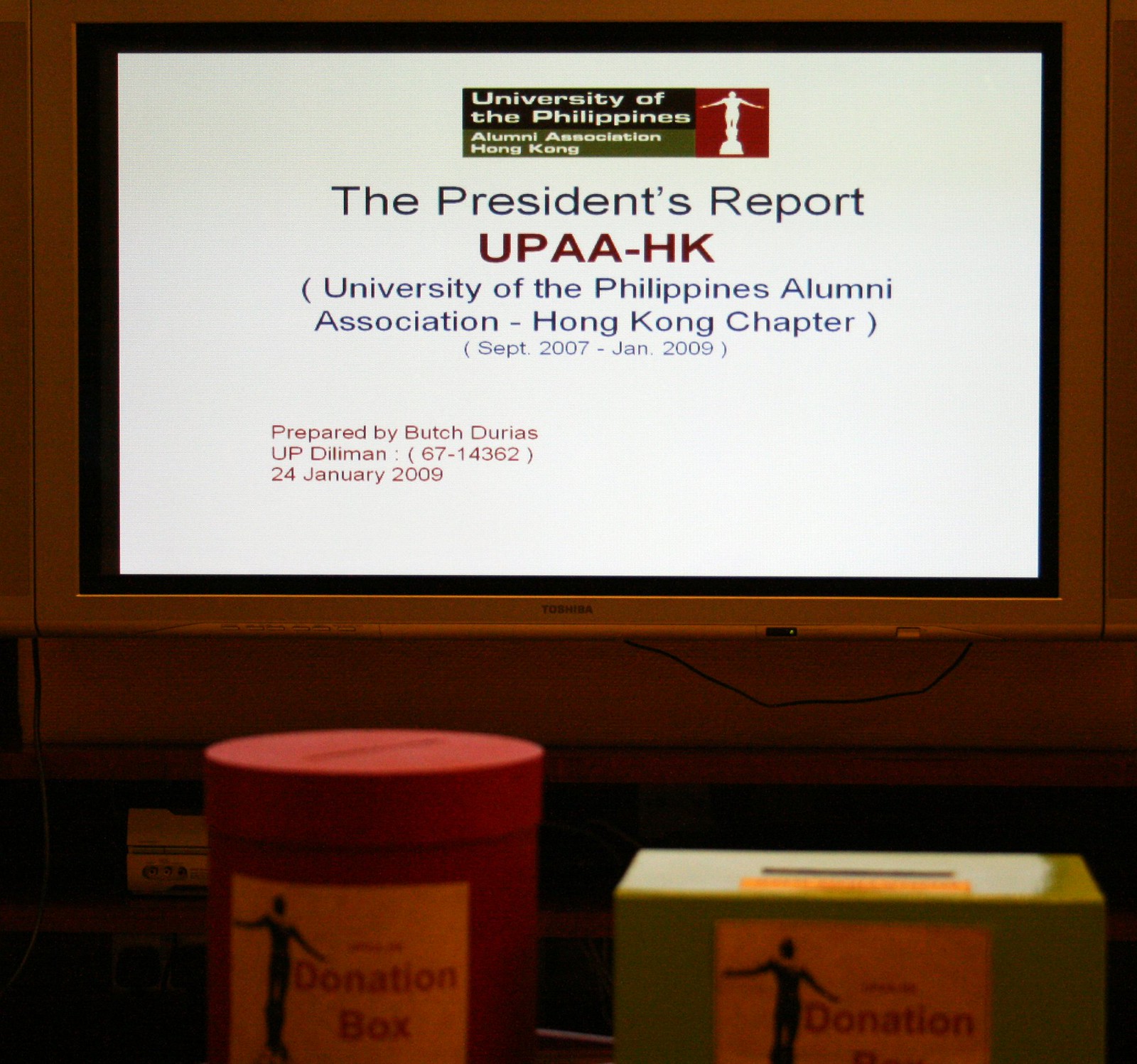The image depicts a TV screen mounted on a wall, displaying informational content characteristic of a conference setting. The screen has a white background with predominantly blue and red text and features the emblem of the University of the Philippines and the Alumni Association of Hong Kong. The title "President's Report" is prominently displayed along with details such as “University of the Philippines Alumni Association Hong Kong Chapter (UPAA-HK).” Dates specified range from September 2007 to January 2009. The presentation was prepared by Butch Dorez of UP Diliman, with his ID number 6714362, and the date noted as January 24, 2009. In the foreground, there are two donation boxes: a red cylindrical box with a slot on top, and a green rectangular box, also with a slot on top. Both boxes bear stickers depicting a silhouette of a person and the label "donation box." The image suggests a meeting or presentation event for the University of the Philippines Alumni Association in Hong Kong, documenting past activities and financial contributions.